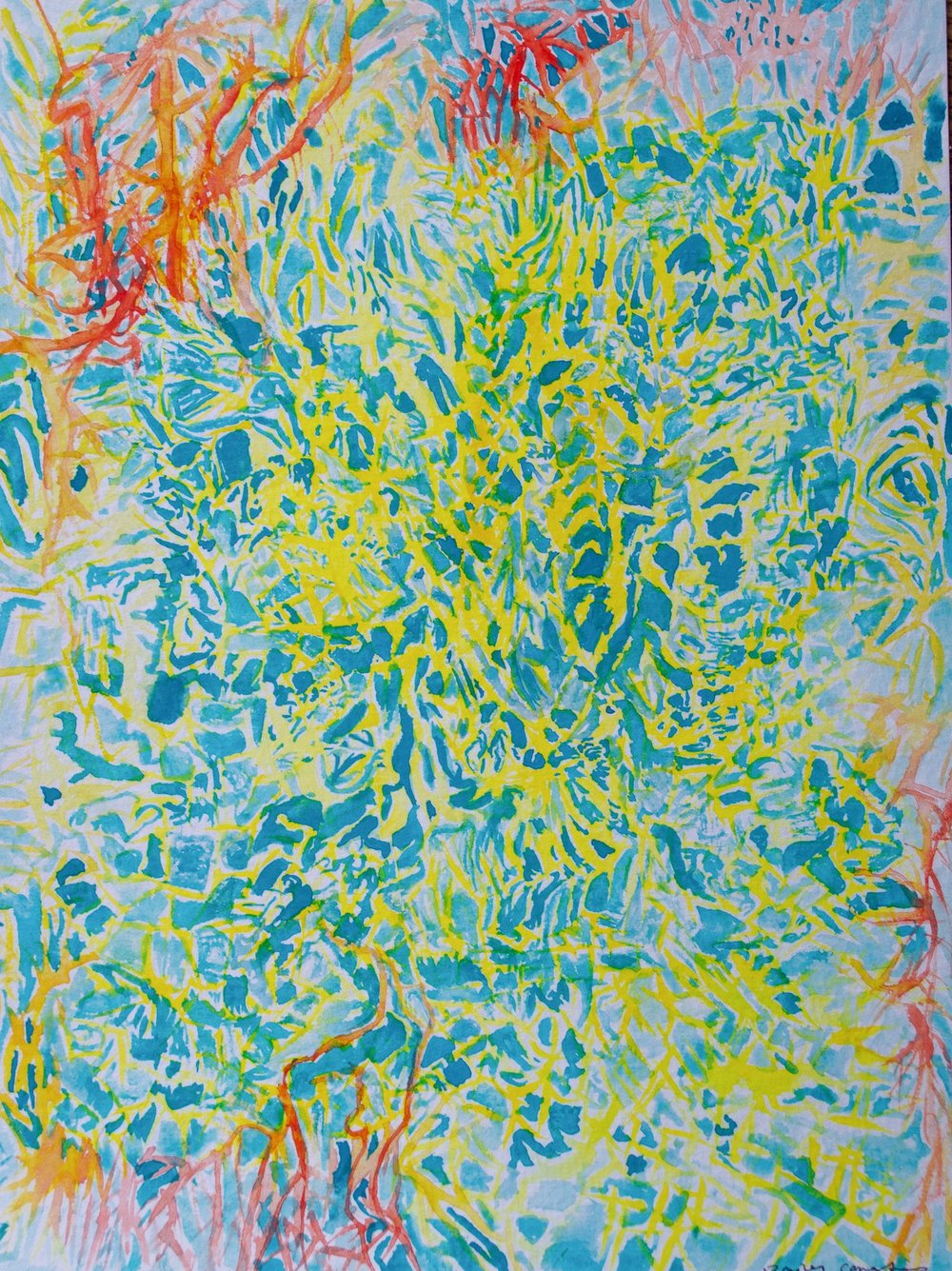This modern and abstract painting features a complex interplay of colors and lines set against a white canvas. Dominating the center are vibrant yellow lines interwoven with hues of blue and green, creating an intricate focal point. Surrounding this central chaos, the edges of the painting showcase vivid red, orange, and pink lines, particularly concentrated in the top left and right corners, as well as the bottom right and left sections. These lines, described as squiggly and veiny, merge and swirl together without forming any recognizable shapes, contributing to the overall abstract and meaningless nature of the artwork. The painting lacks a visible signature, further emphasizing its enigmatic quality.